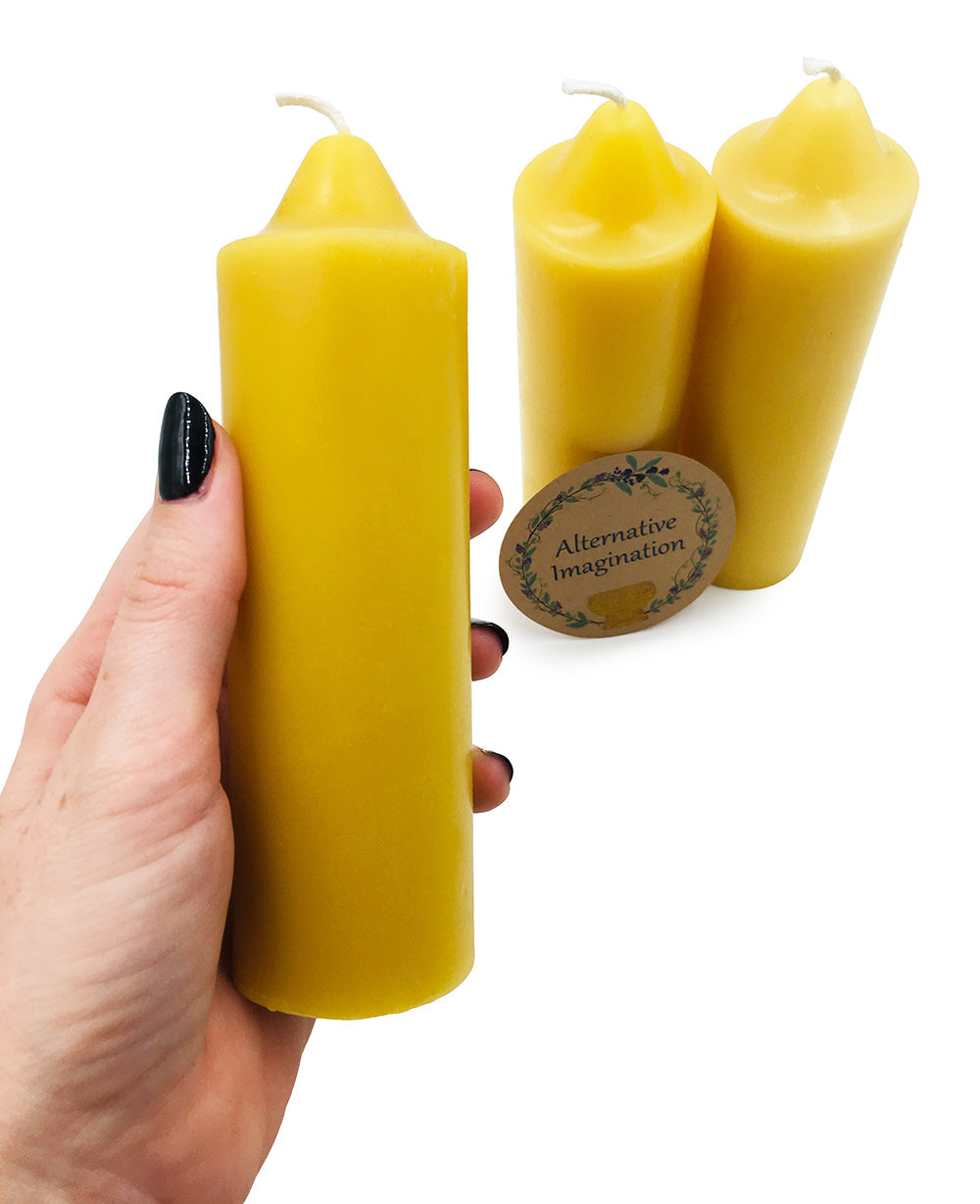The image features a plain white background with no visible borders. In the lower left corner, a Caucasian female hand is prominently displayed, its wrist and the back of the hand forming a border line. Her fingernails are painted black, and she is holding a cylindrical yellow beeswax candle that is about three inches high and an inch wide. The candle has a domed top with a small white wick protruding from it.

In the background, there are two more candles standing side by side, slightly tilted forward, giving the illusion that they are suspended in the air. Both candles are wrapped in cellophane, suggesting they are sold as a set. Positioned in front of the left candle is a brown circle, seemingly cut out from brown cardstock. This circle features a ring of ivy with purple flowers and green leaves, with the words "Alternative Imagination" printed in black in the center. At the bottom of this arrangement, there is a small golden goblet.